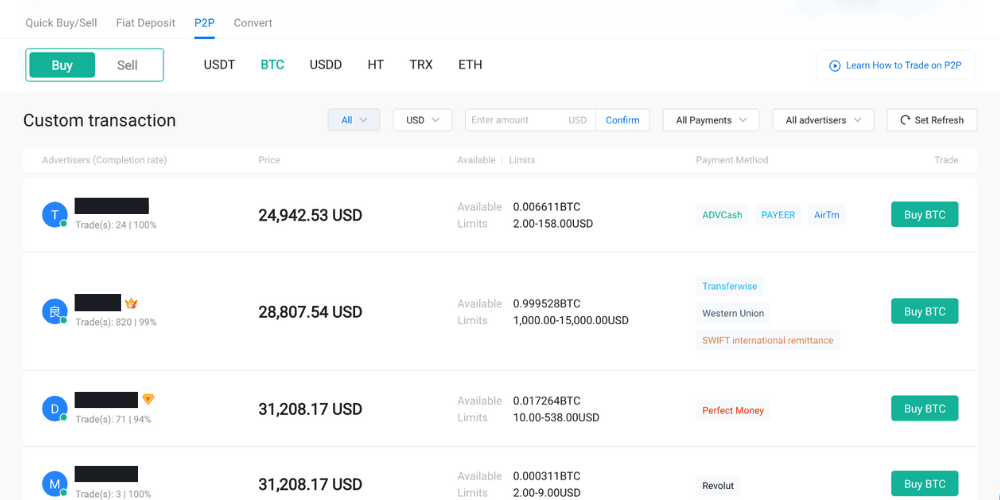The image features a user interface with a light blue background. At the top, there are several navigation options including "Quick Buy/Sell," "Fiat Deposit," and "P2P," which is underlined in blue. To the right, there's a blue circular icon with an arrow that says "Learn How to Trade in P2P."

Below these options, there's a prominent green button with "Buy" in white text. Adjacent to it is a white button with "Sell." Key cryptocurrencies are listed in blue, such as USDT, BTC, USDD, HT, TRX, and ETH. Additionally, a blue link labeled "Custom Transaction" stands out among the menu items.

Further down, there are multiple buttons including "All" with a down arrow beside "USD," and a confirm button along with "All Payments" and "All Advertisers" buttons. There's an option to "Set Refresh" as well.

The central section contains a large white box. Inside, there’s a blue circle with a "T" in it, alongside another smaller blue circle at the bottom. Following this, a figure "24,942.53 USD" is displayed in black text with some accompanying numbers. Below, terms like "Advance Cash," "Pay For," and "Active" are visible. There are also green "Buy BTC" buttons alongside these details.

Additionally, there's an entry marked with a blue circle containing a white icon, obscured details, and "28,807.54 USD" in black text. Several more numbers and icons in blue, purple, and pink follow, alongside another green "Buy BTC" button.

Further listings show blue circles with a "D" or an "M," blacked-out amounts like "31,208.17 USD," and payment options such as "Perfect Money" and "Revolt" in pink. Each of these entries also includes a green "Buy BTC" button.

This interface appears to be a detailed overview of a cryptocurrency trading platform, featuring various payment options, transaction details, and purchase buttons.